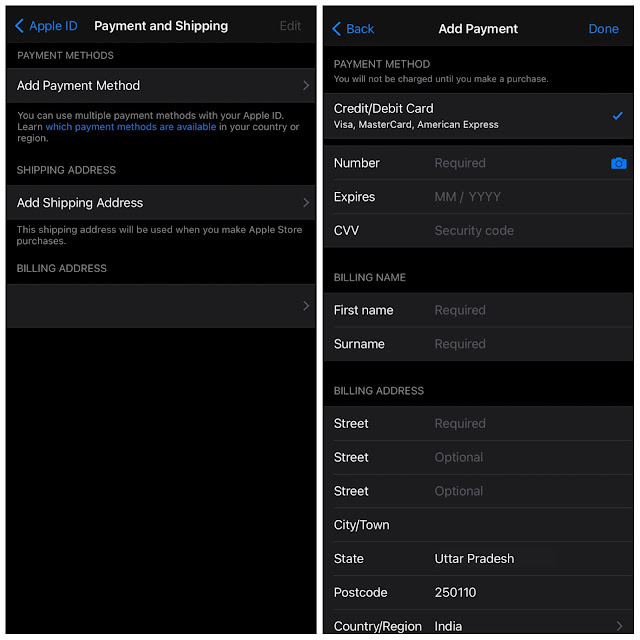**Title: Apple ID Payment and Shipping Details Setup**

**Image Description:**

The image displays two black screens side by side, portraying the setup process for Apple ID payment and shipping details. 

- **Left Screen:**
  - The top section features “Apple ID” in blue with a left-pointing arrow, indicating navigation.
  - Below it, the section titled "Payment & Shipping" is displayed in white text.
  - **Payment Methods:** 
    - A box labeled "Add Payment Method" is present.
    - An informational note states, “You can use multiple payment methods with your Apple ID. Learn which payment methods are available in your country or region.”
  - **Shipping Address:**
    - A button labeled "Add Shipping Address" is accompanied by a right-pointing arrow.
    - A description explains, "This shipping address will be used when you make Apple Store purchases."
  - **Billing Address:**
    - There is a box with a right-pointing arrow to possibly add or edit the billing address.

- **Right Screen:**
  - At the top, the word "Back" in blue with a left-pointing arrow indicates a navigational option.
  - The title "Add Payment" appears in white, followed by a "Done" button in blue.
  - **Payment Method:**
    - An assurance message states, “You will not be charged until you make a purchase.”
    - Below, options for credit and debit cards including Visa, MasterCard, and American Express are shown, with a blue checkmark next to the accepted cards.
    - Fields for required entry include:
      - **Card Information:**
        - “Number” with a blue camera icon for scanning the card.
        - “Expires” with month and year entry.
        - “CVV” for the security code.
      - **Billing Name:**
        - Fields for "First Name" and "Surname," both marked as required.
      - **Billing Address:**
        - "Street" marked as required.
        - Fields for "Street 2" and "Street 3" are optional.
        - Fields for "City / Town", "State," with an example "Uttar Pradesh," "Postcode" stated as "250110," and "Country / Region" as "India."

This detailed depiction helps in understanding the various fields and steps involved in setting up payment and shipping options for an Apple ID.